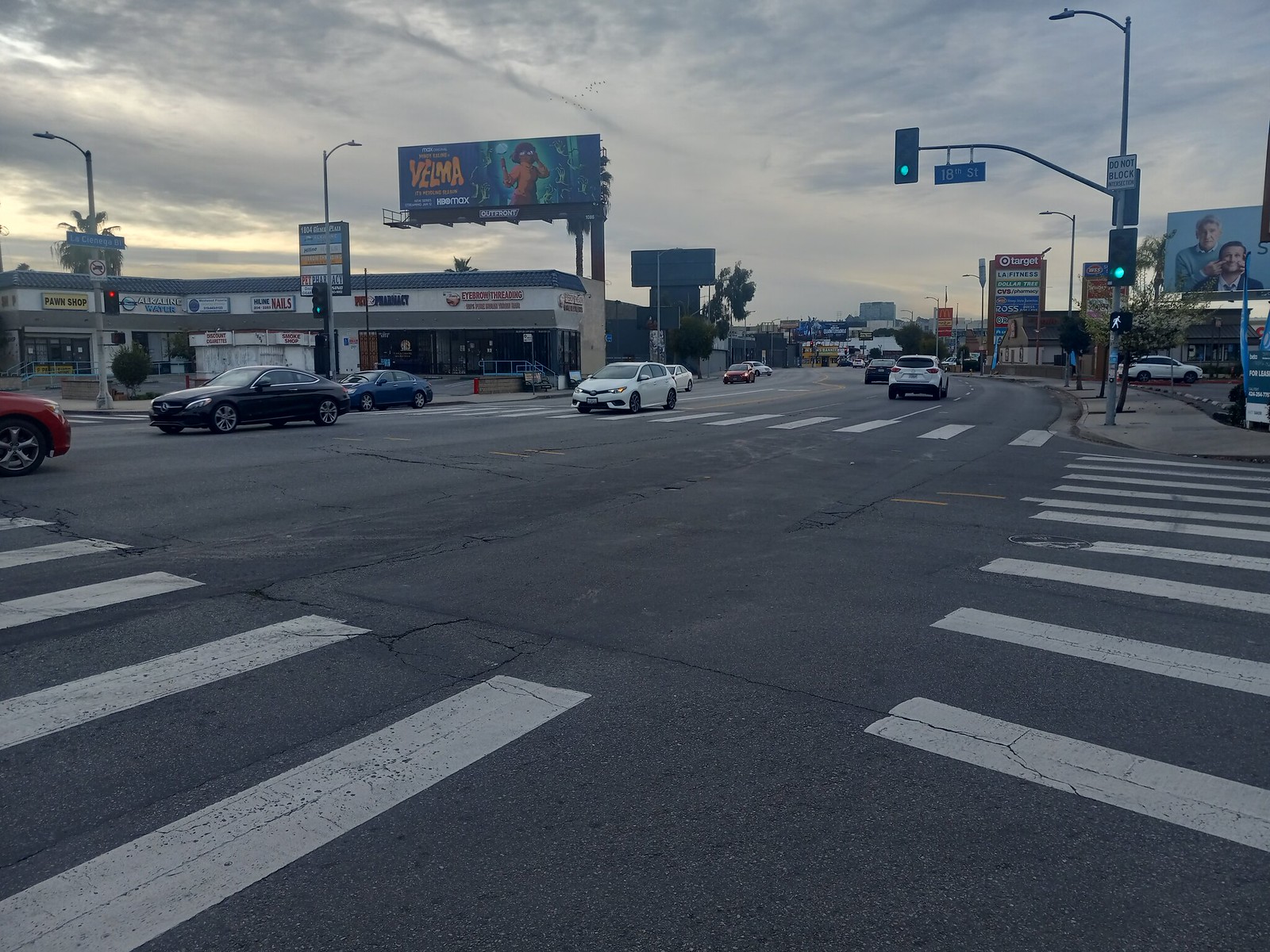This detailed image depicts a bustling urban intersection viewed from a corner sidewalk. At the four-way stoplight, a total of approximately ten cars are visible, including some in the distant background, traversing the middle lanes. Directly ahead and extending to the left and right are white crosswalk lines. Across the street to the left side is an outlet mall with several stores, although the store names are indistinguishable. Above the stores looms a giant billboard featuring Velma from Scooby-Doo, seemingly underwater, surrounded by seaweed and a blue background. Elevated above the stores, two palm trees frame the scene—one to the left and another to the right. The overcast sky is grayish, with a hint of sunset light visible on the left, suggesting the sun is setting. On the right side of the street, another billboard shows two individuals, with one appearing to touch the other's face. In the background, a series of buildings and stores stretch further down the street, adding to the urban depth of the view.